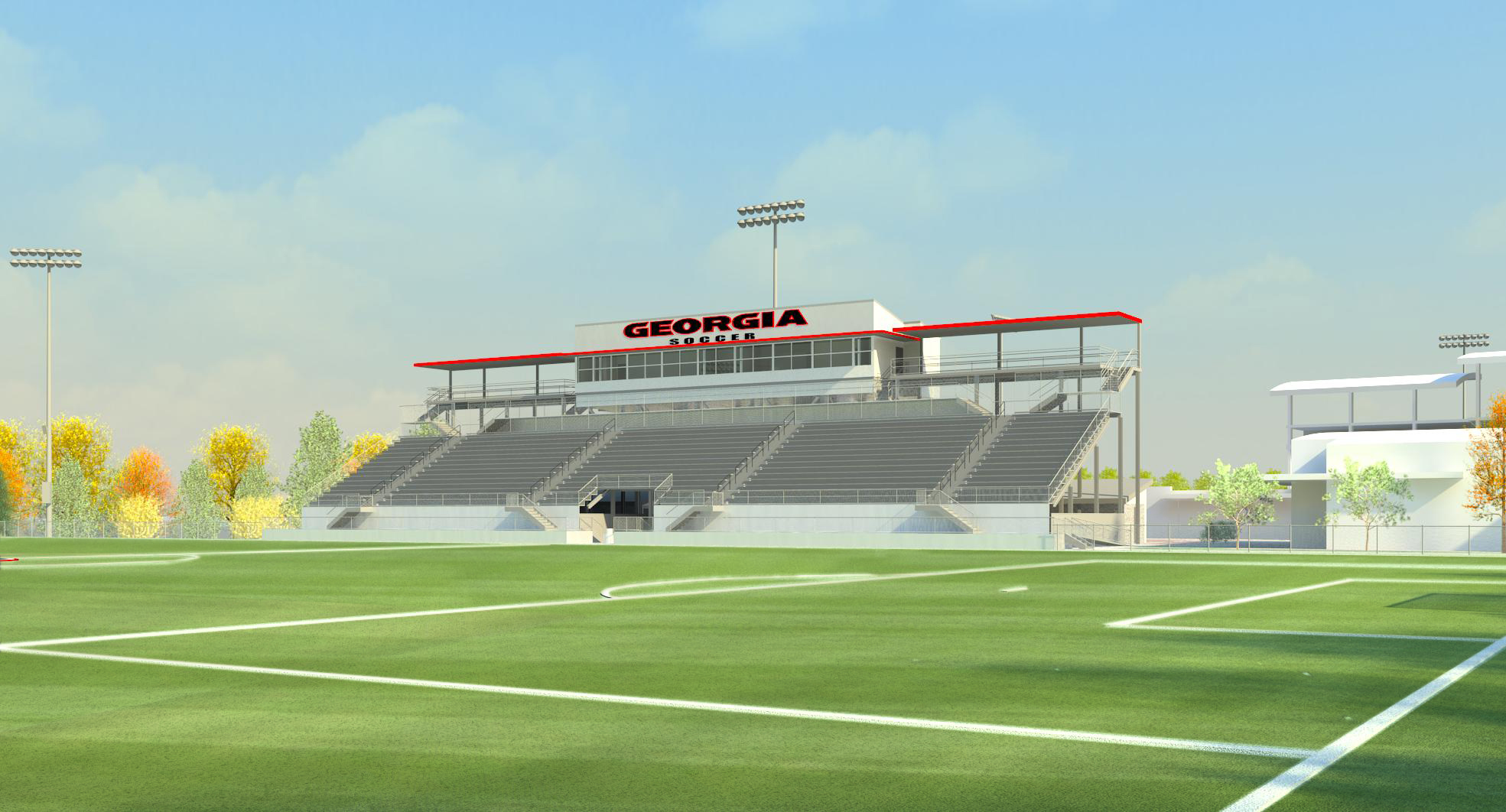This image is a detailed, computer-generated, 3D digital rendering of a soccer stadium. The view is from one corner of the green grass field, marked with white lines delineating the boundaries, midline, and goalie areas typical of a soccer field. Directly across the field stands a large, elevated stadium seating area with inclined rows of benches, designed in a bleacher-style. At the top of these stands is an enclosed, long white booth, likely intended for sports announcers and officials, which prominently displays the words "Georgia Soccer" in black letters outlined in red. In the background, there are tall stadium lights meant to illuminate the field, trees lining the horizon, and a white building on the right side, possibly part of the sports complex. The scene is set under a sky with wispy white clouds, reinforcing that this is not a photorealistic image but an architect's colored rendering of a proposed soccer stadium.